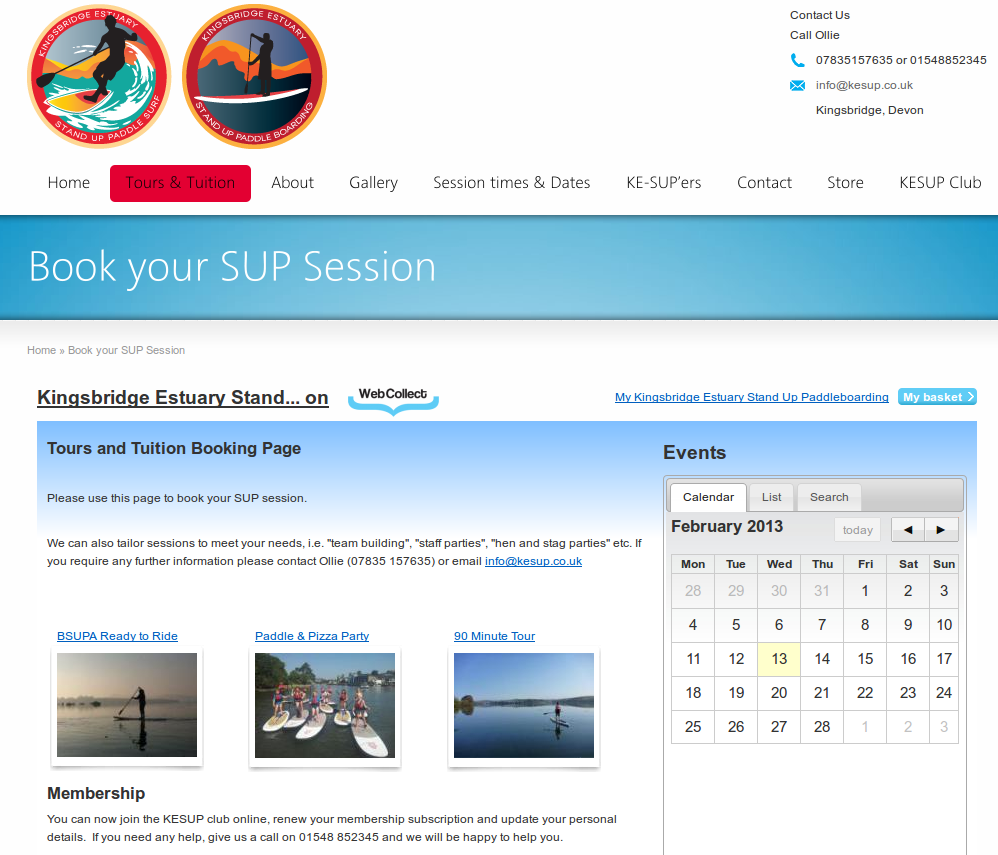A man is standing on a paddleboard, waveboarding with a paddle. To his right, there is an icon showing a person on a paddleboard, moving the paddle but without waves. Below that, there are several navigation tabs: Home, Tourist Intuition (highlighted in a red box), About, Gallery, Session Times and Dates, KE-SUPers, Contacts, or KESUP Club. 

At the top right, contact details are provided: "Contact Us, Call Ollie at 07835-157-635 or 15488-52345, info@kesup.co.uk, Kingsbridge, Devon." Below the tabs, a prominent blue bar reads, "Book Your SUP Session." 

Underneath, the header "Kingsbridge Estuary Stand-On Web Collect Tourist Intuition Booking Page" invites visitors to book a SUP session. The page features actual photographs: one of a man standing alone on the water, another of a group of around six people on paddleboards, and a third of a man on a lake, appearing small due to the distance.

To the right of the images, there is an events calendar showing February 2013, with the current date being the 13th.